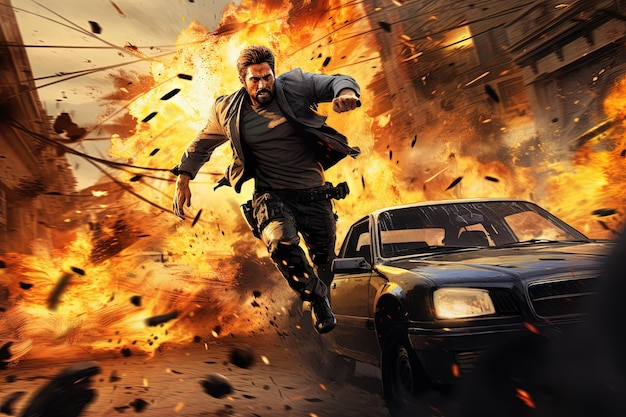The image appears to be a dramatic scene from an action movie or a highly realistic video game. At the center, a distressed man is captured in mid-air, seemingly propelled forward by a massive explosion behind him. He is dressed in black pants, black boots, a gray t-shirt, a black jacket, and a gun holster strapped to his belt or leg, emphasizing his role as an action hero. The man has a full head of hair, along with a mustache and beard; one hand is clenched in a fist while the other is extended backward, reflecting his dynamic movement. The explosion behind him engulfs several buildings in a fiery ball of orange, yellow, and red hues, sending shrapnel and debris flying in all directions. To his left, a black sedan with its headlights on sits on the pavement, possibly from the 70s or 80s, with its windows appearing scratched or melting due to the intense heat. The chaotic backdrop, complete with collapsing power lines, enhances the high-stakes atmosphere of the scene.